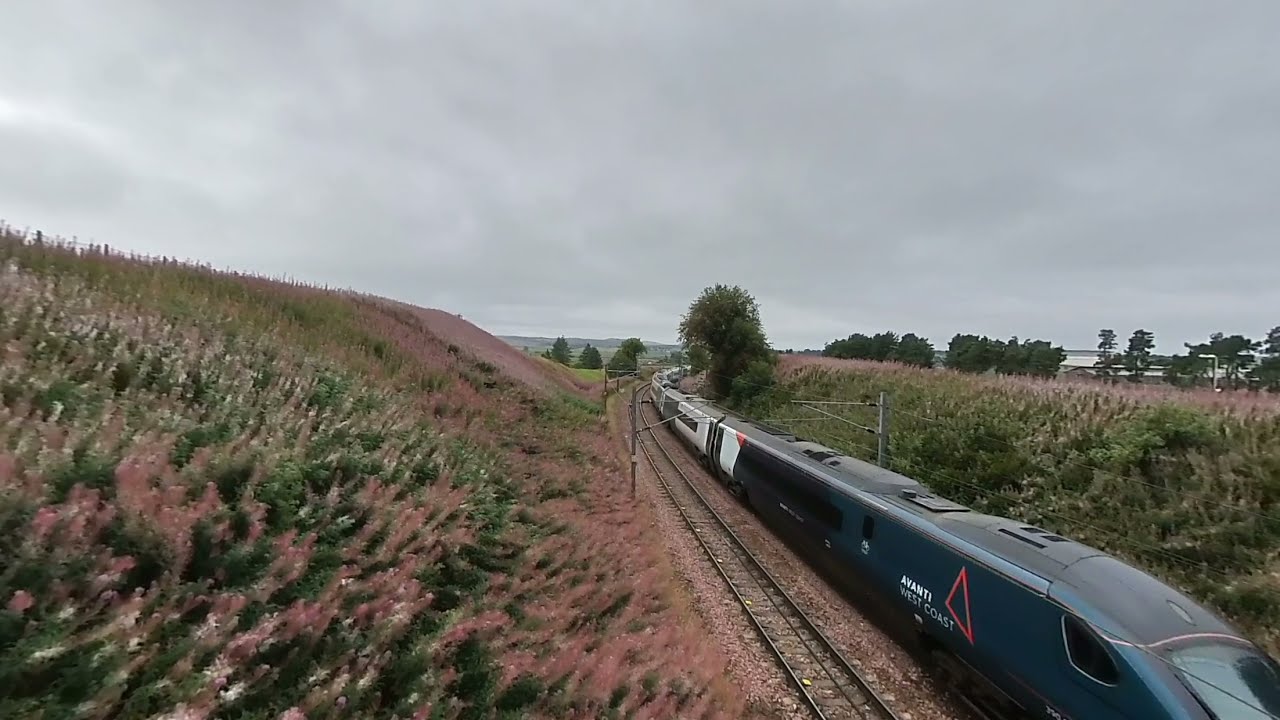The photograph captures an outdoor scene during the daytime, featuring an overcast sky filled with storm clouds. The central focus of the image is a blue Aventi West Coast train with white passenger cars, making its way along a curving track that runs through a rural area. The train is situated on the second set of double tracks, the first set of which remains empty. The tracks appear to lie within a gentle ravine and are flanked by lush, brush-like vegetation that is green, pinkish-red, and white in color, resembling feather-like plants. On the left side of the train, a hillside slopes downwards, covered in this distinct flora, while the right side mirrors this with additional vegetation and trees. Further into the background, near the right-hand side, a building peeks out from behind the trees. Off in the distance, faint outlines of mountains are visible beneath the cloudy sky, adding depth to this tranquil rural landscape.